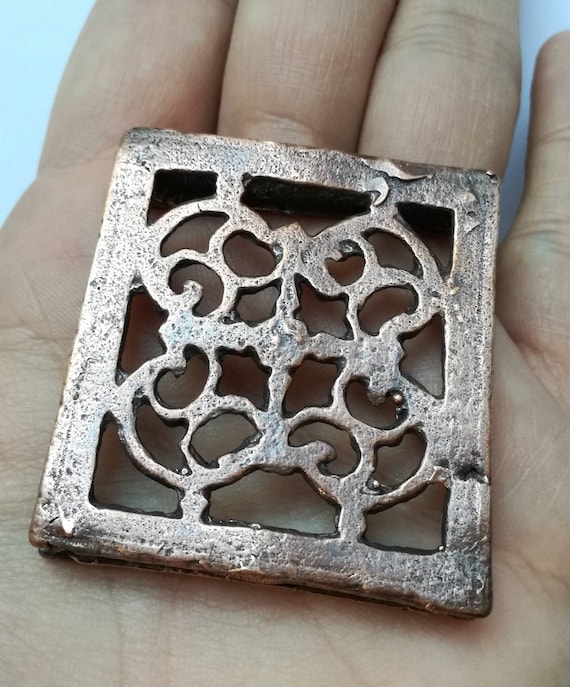This horizontally-aligned photograph showcases a close-up of a weathered male hand, likely belonging to someone around 40 years old, with light brown, somewhat tan skin. The image is taken against a background featuring two shades of light blue, with one shade visible in the upper left corner and the other peeking through the gaps between the fingers. 

The hand is holding a small, horizontally-aligned, rectangular piece of ornate metal, appearing somewhat flat and lying at a diagonal with the top tilting to the right. The metal, with a weathered and tarnished silver or shiny copper color, exhibits signs of age, including ground-in dirt, pitting, and blackened areas. About 1 centimeter in width along the right and left sides, the piece features skinnier edges on the top.

Intricate in design, the metal has a detailed filigree pattern, with arcs emerging towards each corner, where they form two lobes or wing-like shapes, giving an impression of a butterfly, albeit possibly coincidental. This complex network of interconnecting branches is symmetrically arranged with a rough and bumpy main line running through the middle. Perpendicular to this line, a cross-like pattern is evident, adding to the symmetry.

In the center of the metal piece, there are round areas at each corner, housing star-like elongated shapes with circular holes and half-circle curves inside them. The entire structure seems reminiscent of an archaeological relic, hinting at its historical and perhaps cultural significance.